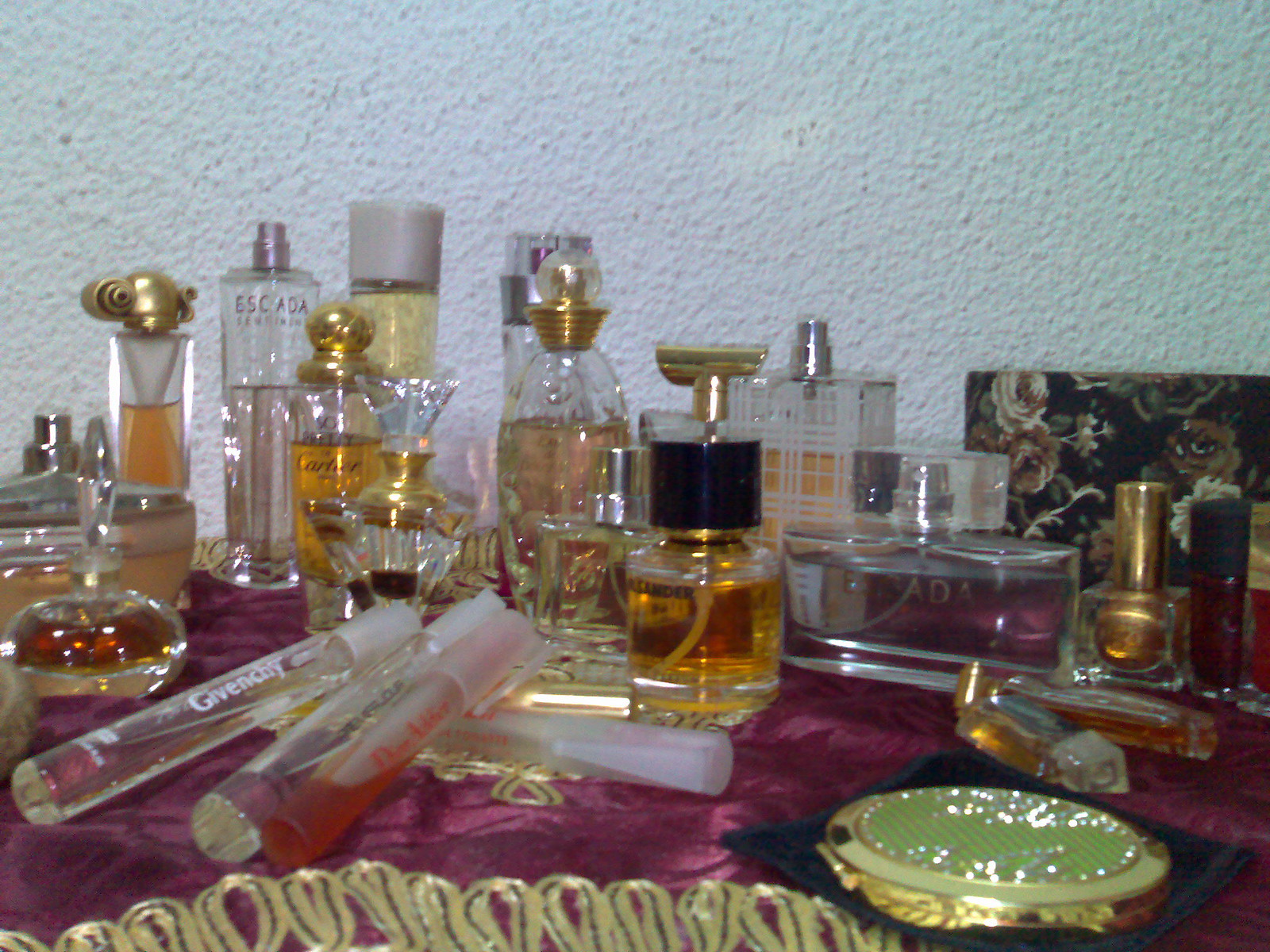The photograph showcases an opulent perfume collection meticulously arranged on a table draped in a luxurious purple velvet cloth. Diverse in size and style, the collection features an array of perfume bottles, from small portable spraying tubes to large desktop jars with atomizers. Notable designer names such as Escada, Cartier, Givenchy, and Prada are visible on the bottles. The shimmering liquids range in color from amber and gold to clear and pink, with some bottles lying on their side, displaying their ornate designs.

Several bottles are topped with an assortment of intricate caps, including gold and white ones, with some lids resembling pieces of intricate jewelry and a particular one resembling a gold knot. One prominent bottle in the foreground has a black lid and contains amber liquid, while another small, mushroom-shaped bottle houses a ruby-colored perfume. A compact mirror is placed at the front, adding to the collection's elegant display. The background features a textured white wall, enhancing the collection's luxurious presentation.